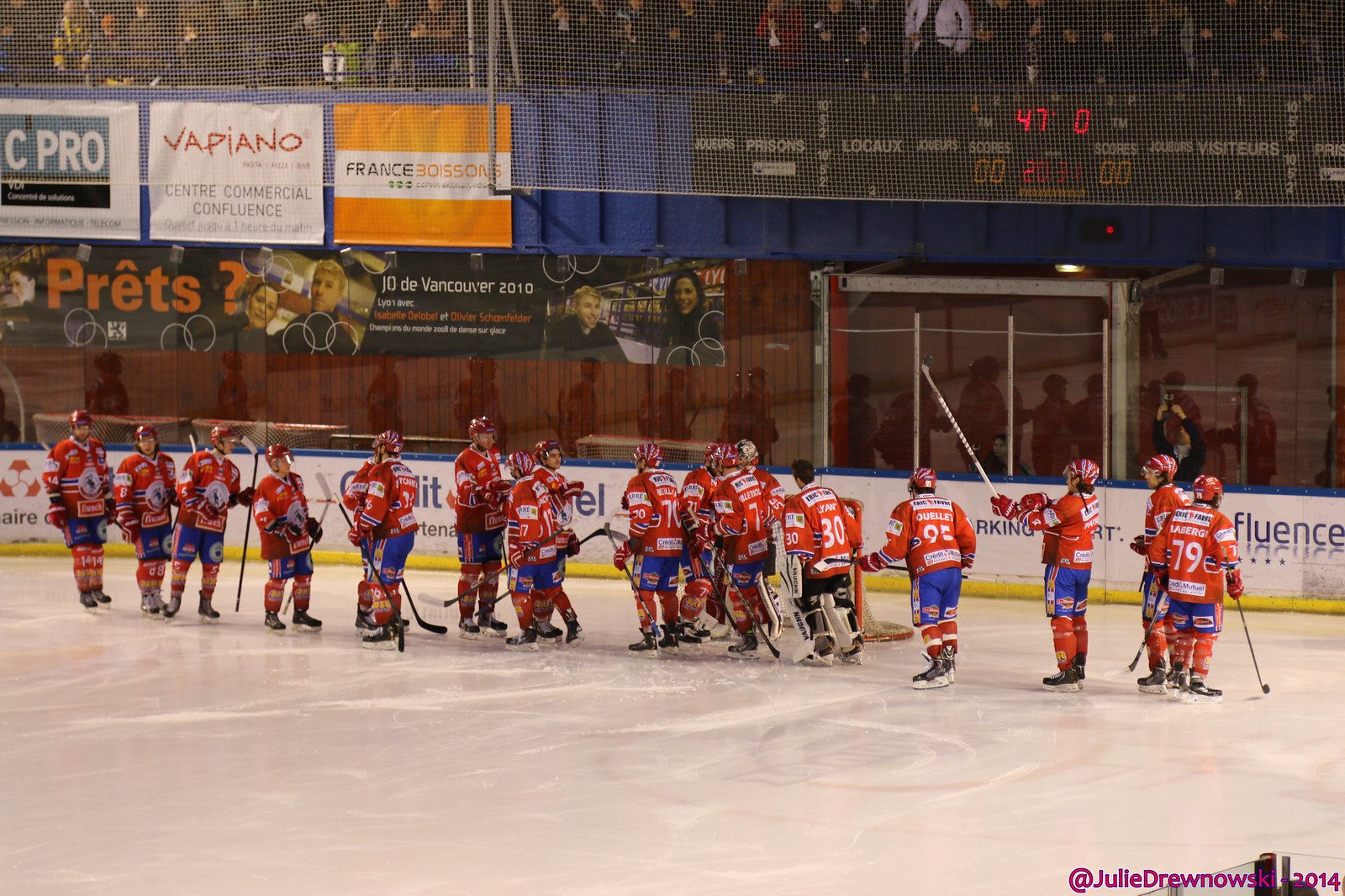This image captures a vibrant scene of an indoor ice hockey game in what appears to be Quebec or Vancouver, indicated by the French-Canadian text and banners in the arena. At the center of the brightly lit, white ice rink, a group of hockey players in red jerseys, red gloves, red helmets, and blue shorts are gathered near the goal, possibly congratulating each other. Their positions form a slightly uneven line, with one player notably not wearing a helmet. Surrounding the rink are clear plexiglass barriers, behind which fans fill the stands. The scoreboard towards the upper right of the image shows a tied score of 0-0, with local (locale) and visitor (visiteurs) teams. Various banners and advertisements, including SeaPro and WebUNO, decorate the scene, adding pops of color such as purple, gray, black, red, blue, orange, and dark blue. The bottom right corner of the image is marked with the photographer's handle: "Julie Jernowski, 2014." Additional details in the glass wall behind the players reveal reflections, security personnel, and a cameraman, enhancing the dynamic and bustling atmosphere of this live event.